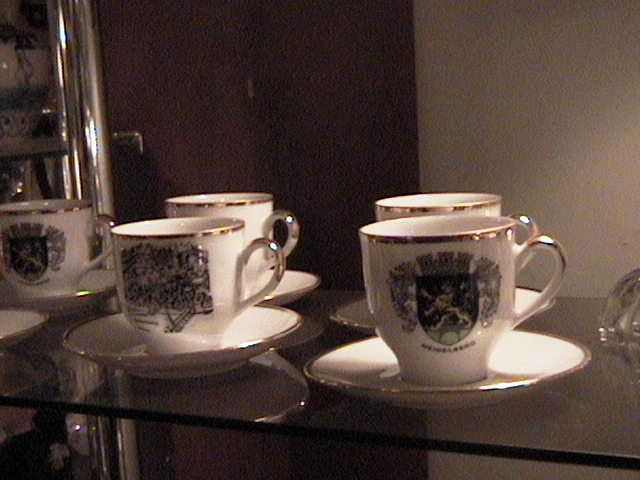The photograph captures the inside of a glass china cabinet, showcasing a collection of five elegant teacups and saucers displayed on a dark brown glass shelf. Each teacup is accompanied by a matching saucer, both in a creamy beige color with intricate gold detailing around the rims and handles, which gleam in the ambient light. The handles of the cups are all positioned facing the right side of the image, while the cups themselves are slightly angled towards the camera, slanting to the left. In the center of each cup, a regal griffin emblem, depicted in brown and green shades, can be seen, resembling a family crest. The detailed embellishments include shields and ornamental designs. The background features a beige wall or cabinet backing, and to the left, a dark brown door with a small gold handle is partially visible. The entire scene exudes a sense of refined elegance and meticulous arrangement, reflective of cherished collectibles on display.